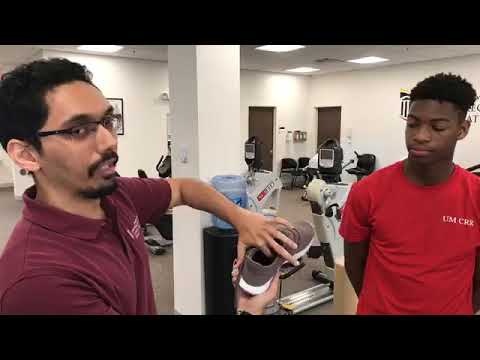In the image, two young men are positioned in what appears to be a low-quality gym or physical rehab center, characterized by the presence of various exercise equipment such as cycle machines in the background. The setting is a white-walled room that might be part of a larger facility.

On the left side of the image, a man of Latino descent is seen holding a brown sneaker and appears to be discussing its features, possibly its support or mechanics. He has short black hair, slightly receding at the forehead, and wears a cranberry-colored, collared short-sleeved pullover shirt. He is looking towards the camera with his index finger placed inside the sneaker, as if explaining something about its interior padding.

To his right stands a young African gentleman in his early 20s, dressed in a red t-shirt with the lettering "UMCRR" on the right breast. He has short, fluffy hair on top and looks towards the man holding the shoe with a slightly sleepy expression, his eyes partially closed. The overall image quality is low, making some details hard to discern, but it's evident that the focus is on the interaction between the two men over the shoe, likely related to some aspect of physical therapy or shoe mechanics.